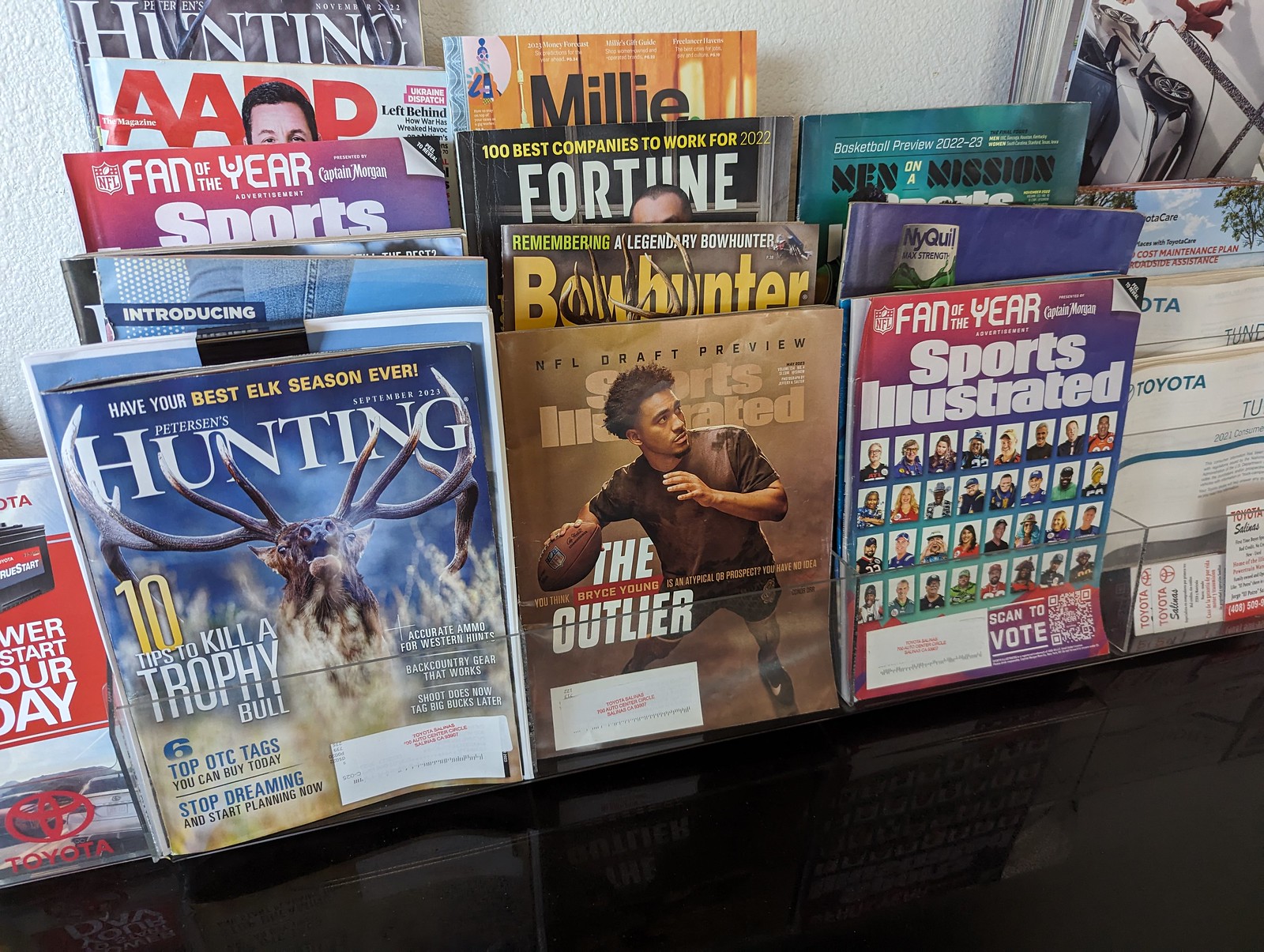This is a color photograph depicting a magazine rack display on a black table, likely situated in a waiting room, possibly of a car dealership. The display features a variety of magazines, including multiple issues of Sports Illustrated, Hunting, Peterson's Hunting, NFL Draft Preview, Bowhunter Magazine, Fortune, Man on a Mission, and the Sports Illustrated Fan of the Year edition. Towards the right side of the rack, there are flyers or business cards for Toyota, suggesting an automotive context. All magazines appear to have mailing labels, indicating they are subscription copies provided for customers' reading while they wait.